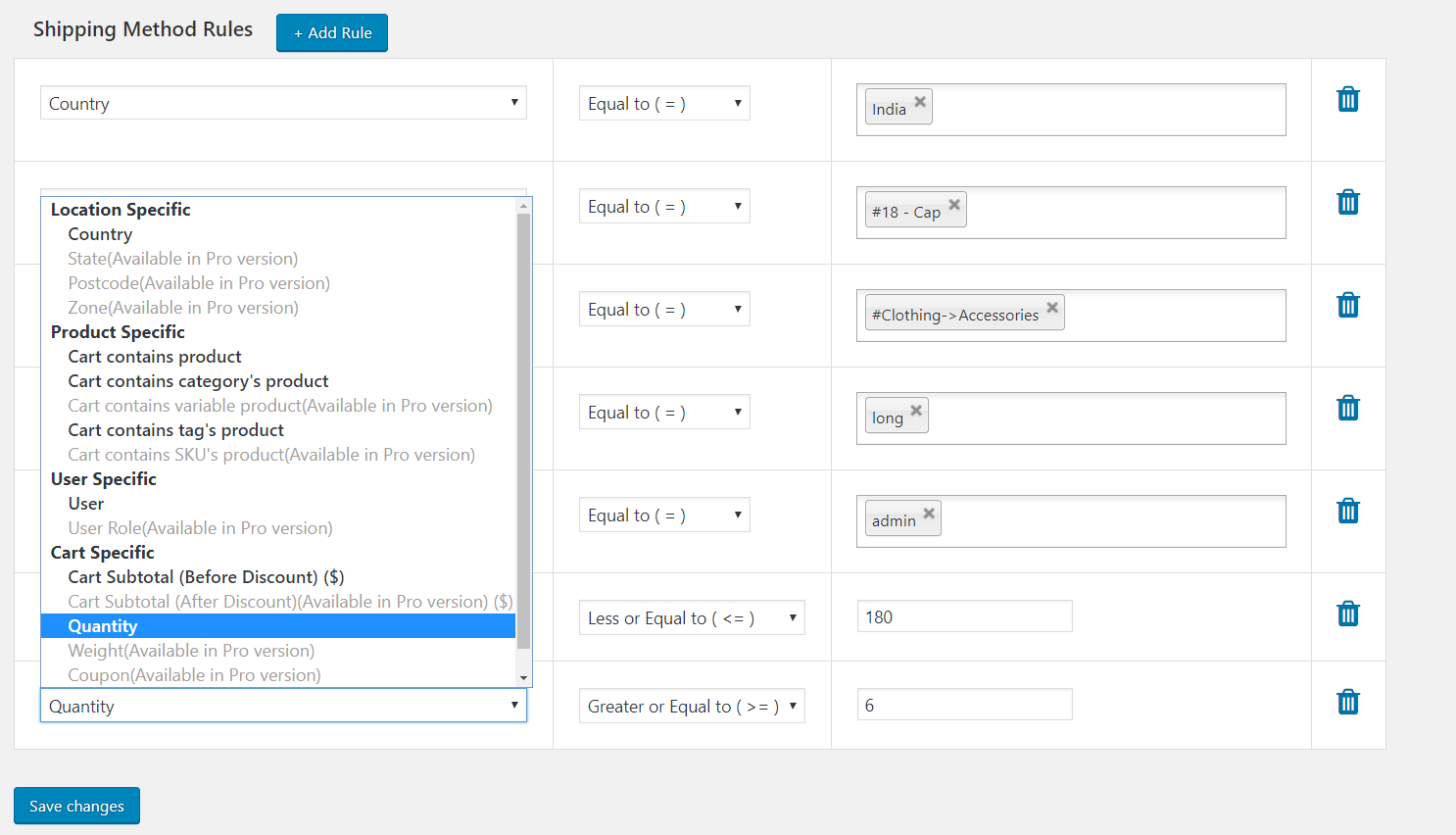The image is a detailed screenshot of a software interface dedicated to configuring shipping method rules. Positioned at the top left corner is a title reading "Shipping Method Rules." Below this, there is a visibly dominant blue box with white text, presumably for emphasizing a section or selected option.

An important feature in the interface includes a dropdown menu labeled "Country," offering the option to filter or select among various countries. Following this, another comprehensive scrollable menu presents several subcategories for specifying conditions: 

- **Location Specific:** Options include Country, State, Postcode, Zone.
- **Product Specific:** Options include Cart Contains Product, Cart Contains Category Product, Cart Contains Variable Product, Cart Contains Tag Product, Cart Contains SKU Product.
- **User Specific:** Options mainly for User and User Role.
- **Cart Specific:** Features such as Cart Subtotal, Cart Subtotal After Discount, Quantity, Weight, Coupon.

Interspersed in the middle of the interface are multiple dropdown menus, each labeled "Equal To" and featuring an equal sign for specifying conditions. This series includes options like "Less or Equal To" and "Greater or Equal To," arranged in a list format.

On the right side of the interface, a specific country entry showing "India" appears, next to which is a trash icon indicating the option to delete this entry if necessary. Further down this section, ambiguous text strings such as "18 cap," "E-Clothing Accessories," "Long," "Administration," "180," and "6" are listed, possibly referencing specific configurations or attributes related to shipping rules.

Finally, at the very bottom left corner of the screenshot, a prominent blue button labeled "Save Changes" is present, facilitating the user to save the configurations made within the interface.